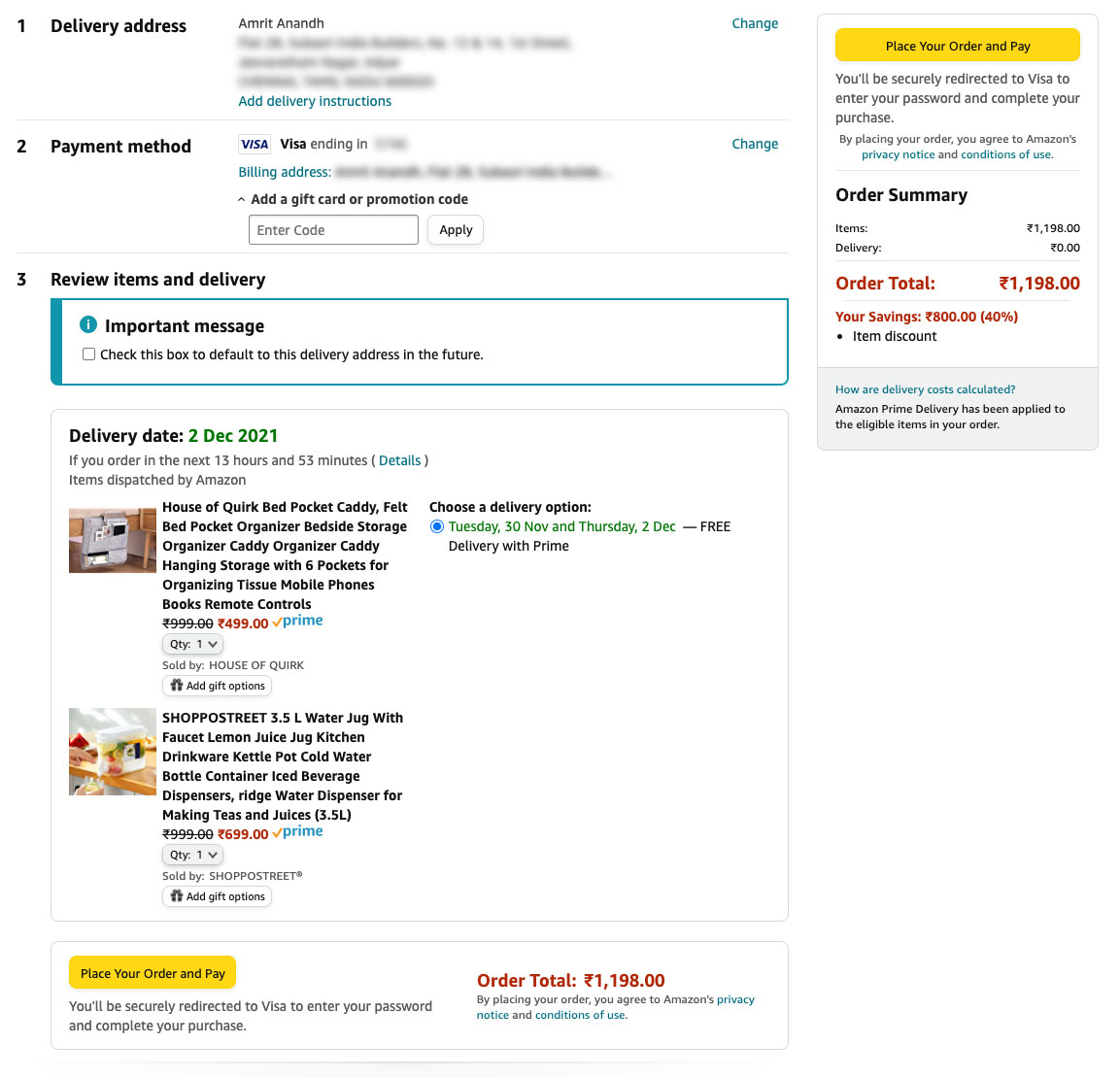The image is a screenshot of an Amazon order page, predominantly featuring a white background with black text. This page indicates an order that is still in progress, not yet completed. At the top, there is a section labeled "1. Delivery Address," which includes the name "Amrit Anand" followed by three lines of blurred-out text, presumably masking the physical address. To the right of this, in blue text, there are options to "Add delivery instructions" and "Change."

Below this is section "2. Payment Method" showcasing the Visa logo and the words "Visa ending in" followed by some blurred-out numbers, disguising the card details. In blue text beneath the payment information, it reads "Billing Address" followed by another blurred-out line, concealing sensitive information. There is also an "Add a gift card or promotion code" field, consisting of a text box labeled "Enter code" accompanied by an "Apply" button.

In section "3. Review Items and Delivery," an important message is highlighted within a blue rectangle: "Check this box to default to this delivery address in the future." Below, the items added to the cart are listed along with their expected delivery date of December 2, 2021. The two items are a "Bed Pocket Caddy" and a "Water Jug."